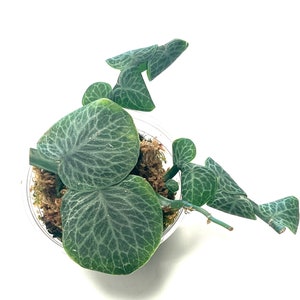The image features a vibrant green plant captured from a top-down perspective. The plant is housed in a white pot, set against a uniformly white background, likely a computer screen, which provides no additional context about its placement indoors or outdoors. The pot reveals brown soil with two prominent central leaves flanked by additional foliage. The large central leaves are marked by distinct white vein patterns, while some of the smaller leaves exhibit triangular shapes. The plant extends outward, with leaves spreading towards the right and top. A faint shadow cast below the pot suggests a light source, adding a subtle depth to the composition.